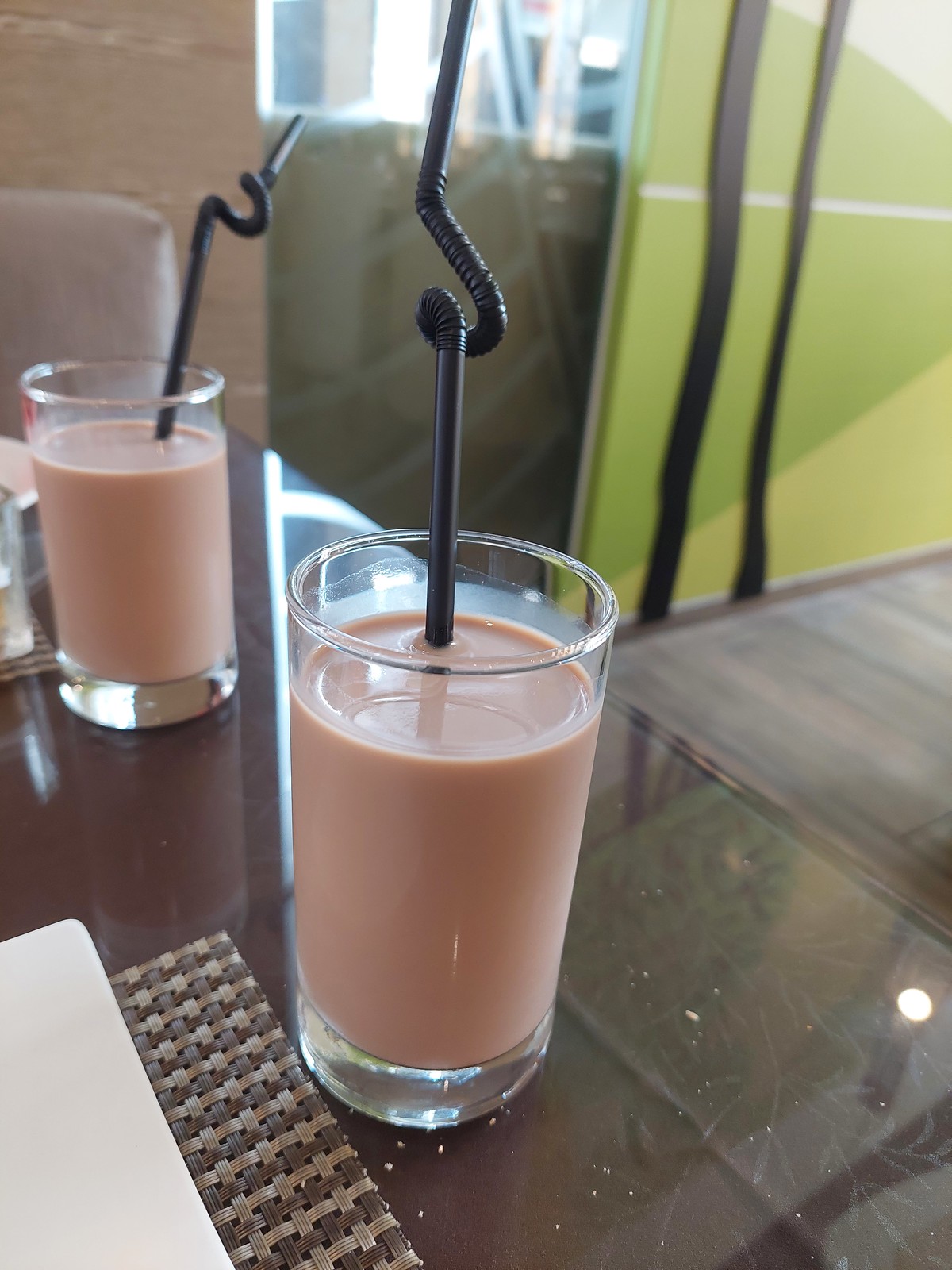In this indoor cafe scene, we see a glass-topped wooden table adorned with two identical clear, cylindrical glasses, each filled with a creamy, medium pinkish-brown beverage suggesting a chocolate milk or smoothie composition. These glasses, with their thick bottoms, house tall, black bendy straws looped stylishly and protruding upward. To the left of the nearer glass rests a light and dark brown woven placemat, and just beneath it, the edge of a white square plate peeks into view. In the backdrop, a lime green wall adds a splash of color, while a gray upholstered chair is partially visible. The ambient natural light filtering through a window softly illuminates the setting, enhancing the inviting, cozy atmosphere of this cafe moment.